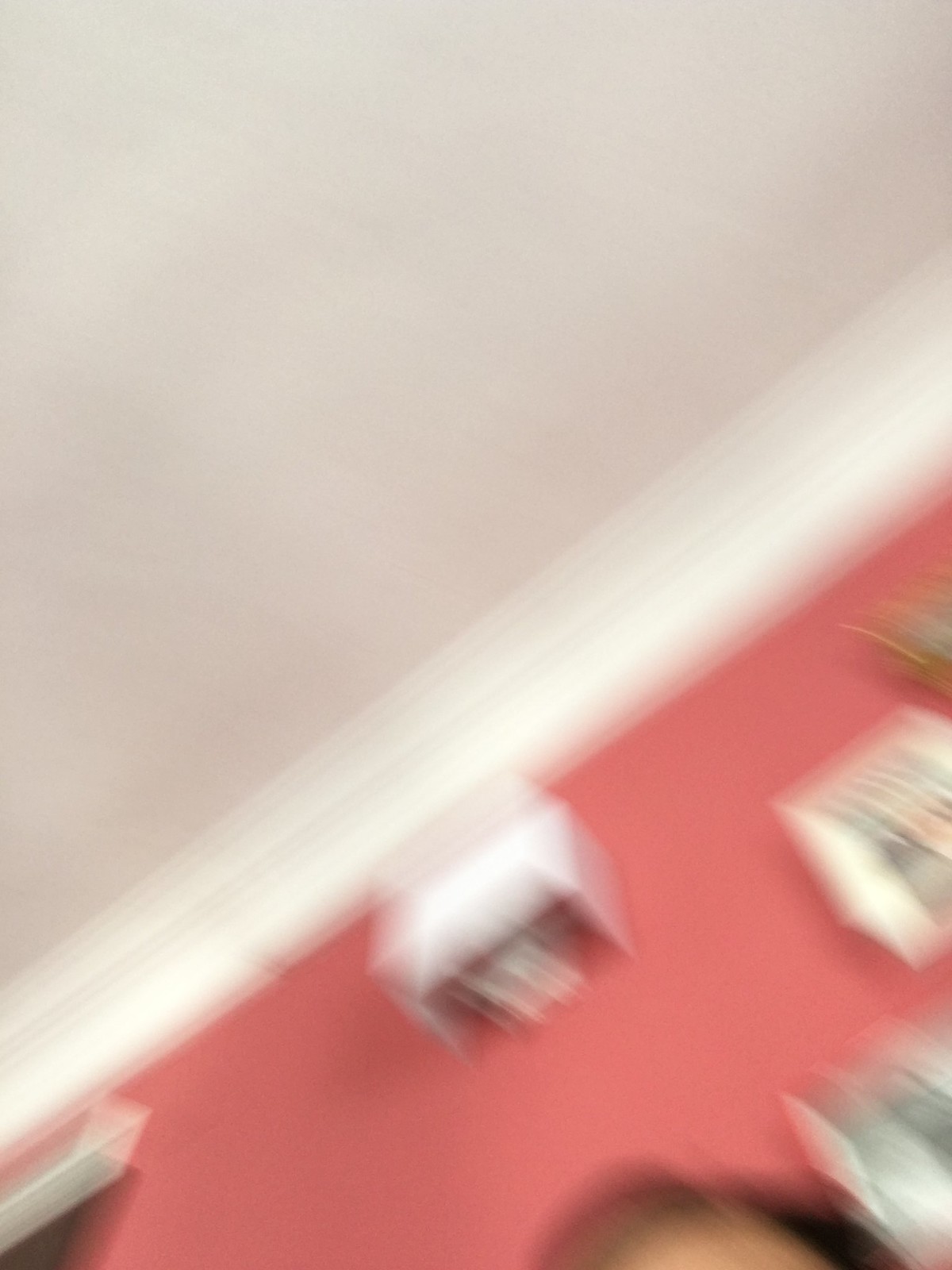This image appears to be a poorly-timed selfie that resulted in a blurred photo. The top of the individual's head is visible in the bottom right corner, indicating movement during the capture. The background reveals a salmon-painted wall adorned with various hangings, which seem to be display boxes, possibly for action figures or other collectibles. There is a white ceiling above, contributing to the indoor setting ambiance. The overall blurriness could suggest either a rapid motion while taking the picture or that it is a still frame extracted from a video clip.